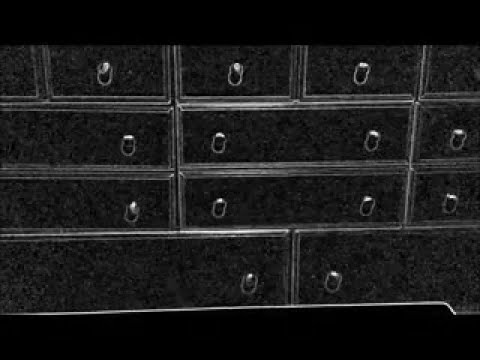The image depicts a stack of black rectangular containers of varying sizes, each adorned with a silver trim and circular silver ports, some containing one and others two. From the bottom level, there are two containers meeting at a central seam, flanked by silver circles. Ascending to the next level, the left-most and right-most boxes display a single silver circle each, while the center box shows two. Higher levels consist of progressively smaller containers, each consistently featuring a single visible silver circle. The overall appearance resembles a series of dresser drawers, with the black top and bottom acting as a plain border. The arrangement creates a visually intriguing pattern with repeated circle motifs, perhaps handles or ports, adding to the industrial aesthetic of the image.